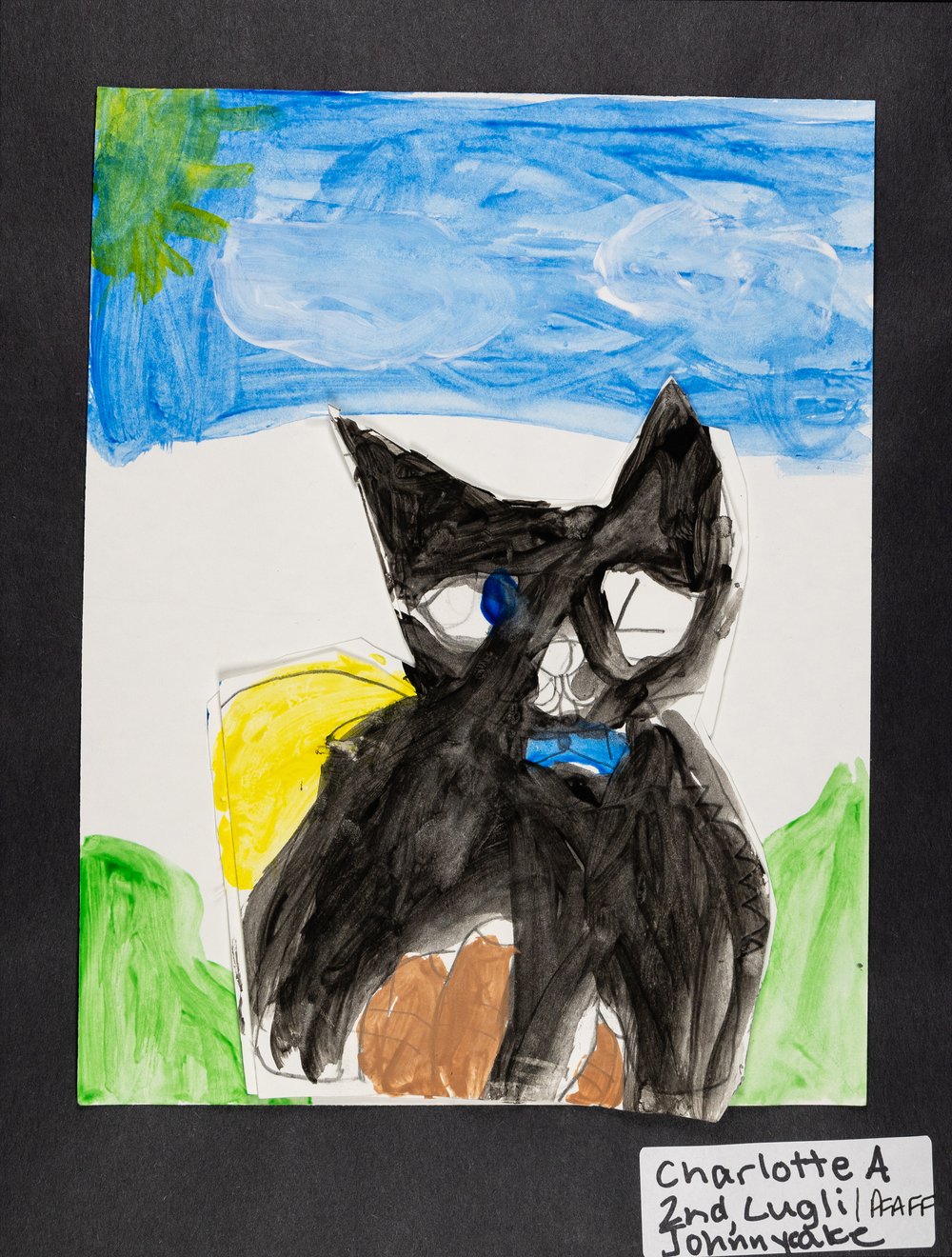The image is a watercolor painting, framed in what appears to be a black or colored flame-like frame. The central focus of the painting is a cat, which has its paws over its eyes. The cat is black with a distinctive blue eye and is depicted wearing a blue tie. It sits on a brown surface, with tufts of green suggesting grass in the bottom corners. The background features a blue sky, with hints of white clouds and a sun that has turned greenish from mixing with the blue. There is some open white space in the middle ground of the sky. An identification tag in the lower right corner reads "Charlotte A. Second, Lugli / Pfaff, and underneath that, Johann Yatce." This adds a personal touch, indicating the artist and possibly the title or series of the painting.